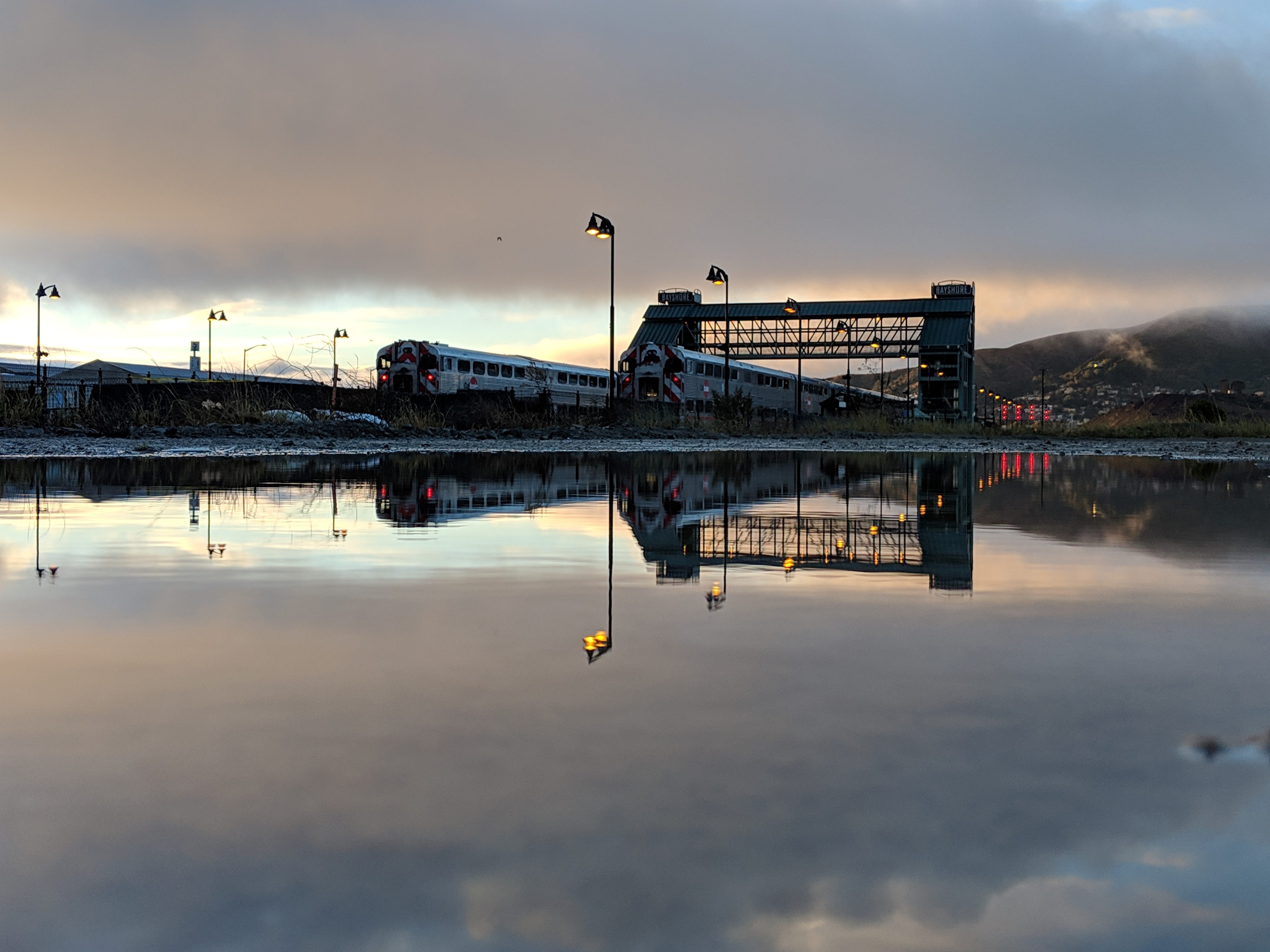The image is a realistic, horizontally oriented photograph likely taken outdoors during the daytime, possibly around dusk given the subdued lighting and cloudy sky. The focus of the image is a calm, reflective body of water, perhaps a lake or a large puddle, occupying the bottom half of the frame. This still water captures a clear reflection of the scene above, doubling the visual elements.

In the central perspective, there are two gray, metal trains parked side by side on train tracks, illuminated by red lights. Alongside these tracks run tall lamp posts, each about 20 to 30 feet high, featuring black frames and glowing with yellow light. A large, metal-framed arched bridge spans over the trains, adding an architectural element to the scene.

To the left of the trains, there are buildings, and in the far background to the right, mountains can be seen, partially obscured by a covering of clouds. Additional lights, possibly from more buildings, are also visible near the mountains, echoing the red glow of the train lights.

In summary, the photograph provides a serene yet detailed depiction of a train station beside a reflective body of water with overcast skies and distant mountainous terrain, featuring trains, a metal bridge, and various light posts that enhance the reflective quality of the water below.